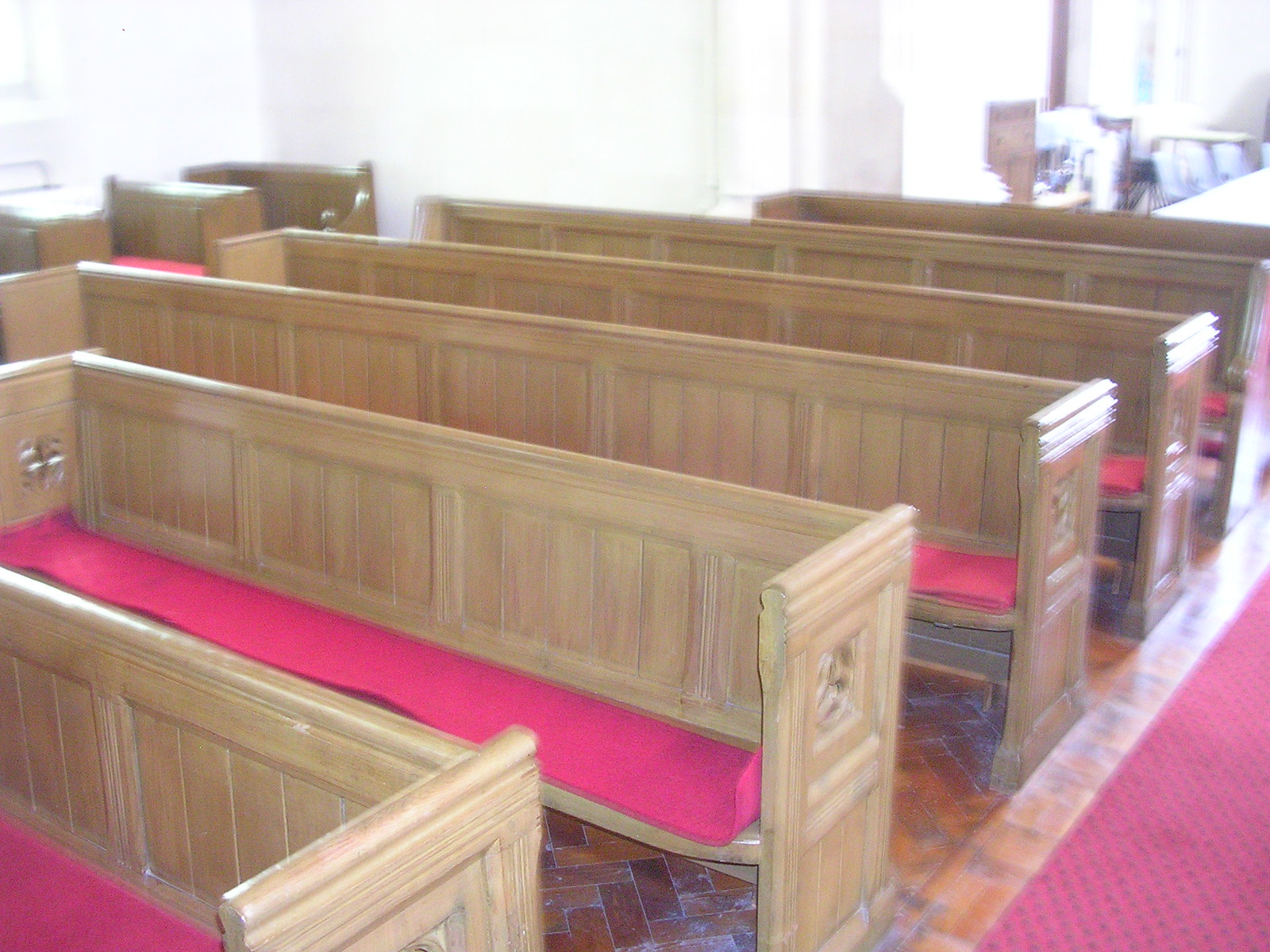This photograph captures a detailed view of a church interior, showcasing a series of six long, rectangular wooden pews arranged diagonally from the lower left to the upper right. The pews, crafted from light maple wood, feature a thin red padding along the entire bench, designed for seating comfort. Each pew has a scroll-like circular design on its sides. Between the rows of pews, a narrow aisle is covered by a red runner carpet, which also lets the brown wood floor peek through in the bottom right corner. Along the left side, against a pristine white wall, small one-seat pews, resembling chairs, can be seen. The bright lighting streaming from the windows casts a vivid glow on the scene, although the photo is slightly out of focus, leading to some blurriness, particularly noticeable in the upper right-hand corner where the image hints at a more intricate, yet undefined structure. The top of the image is bordered by delicate white woodwork, adding an elegant finishing touch to the church's serene atmosphere.